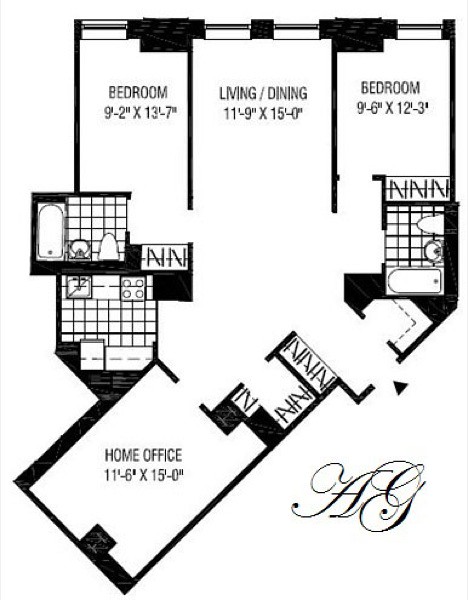This diagram, rendered in black and white, meticulously illustrates the layout of a residential space. In the bottom right corner, an elegant logo consisting of the capital letters "A" and "G" in an italic, cursive style indicates the creator or owner of the building.

At the top of the diagram, three rooms are aligned in a row: the first bedroom, measuring 9 feet 2 inches by 13 feet 7 inches; a combined living and dining area, measuring 11 feet 9 inches by 15 feet; and a second bedroom, measuring 9 feet 6 inches by 12 feet 3 inches. Each of the bedrooms features an adjoining bathroom located below it.

Directly below the left bedroom, there appears to be an unlabeled room which likely represents a kitchen, distinguished by illustrations of a sink and a stovetop. Adjacent to this is a home office space, measuring 11 feet 6 inches by 15 feet, which is connected to a series of closets, suggesting ample storage.